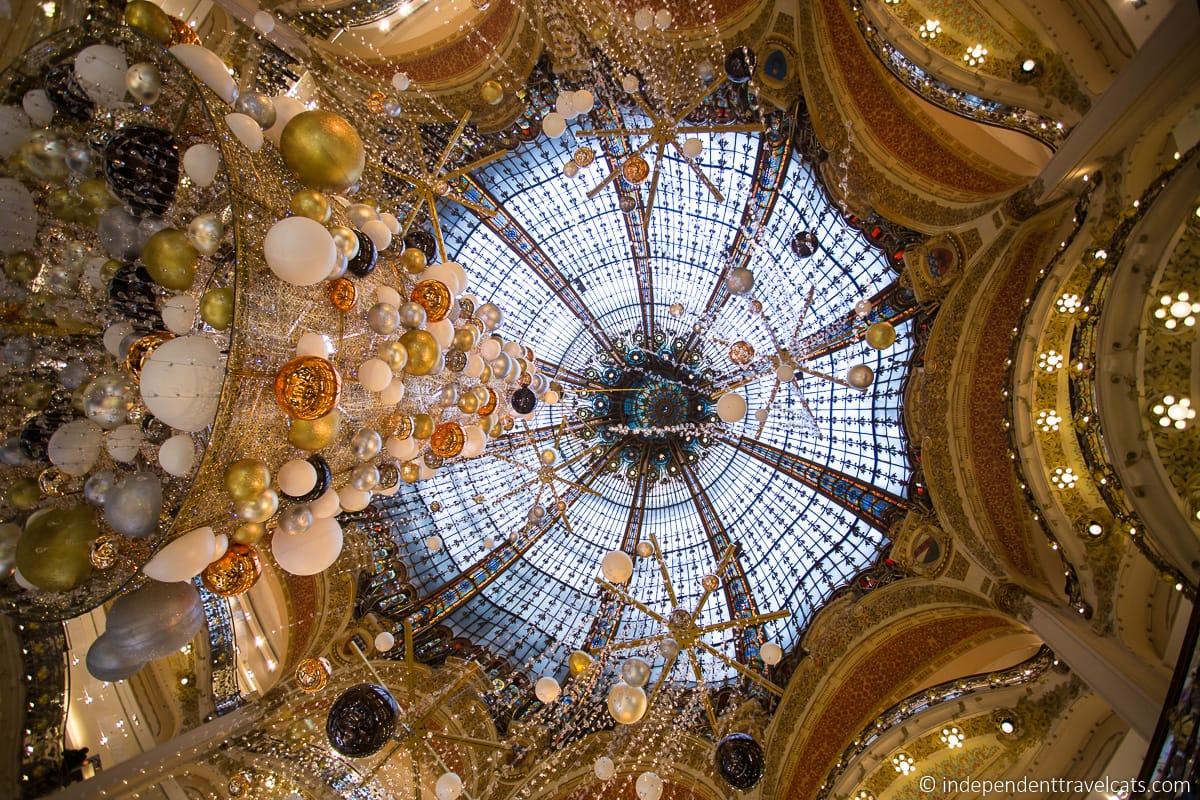The image portrays an ornate interior scene, viewed from the floor looking up towards an opulent glass dome ceiling. The dome is intricately designed, featuring a combination of golden elements and foggy blue glass panels. Surrounding the dome is an octagonal architectural structure adorned with lavish decoration. Hanging from the ceiling are a multitude of objects resembling balloons, crafted in various colors including white, gold, silver, black, and red, arranged in elaborate formations and reminiscent of chandeliers. These "balloons" are suspended by intricate gold chains that appear illuminated and glistening, reflecting the ambient light and adding a sense of grandeur and sparkle to the scene. The setting evokes the atmosphere of a luxurious event, such as a party within a fancy building or cathedral.